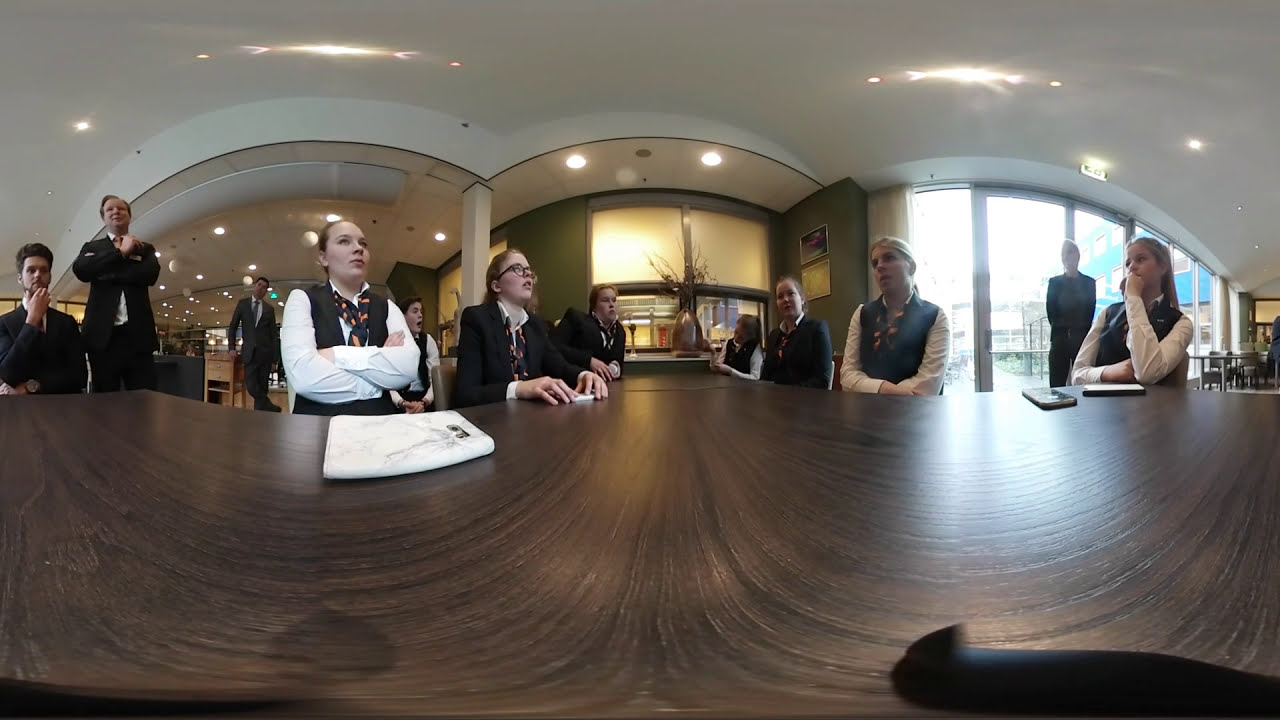The photograph depicts a professional meeting in what appears to be a hotel lobby, given the upscale, elegant setting with recessed accent lighting and expansive windows leading to sliding doors. Seated around a sprawling, brown wooden table are eleven individuals, all dressed in uniform attire. The women wear white, long-sleeved collared shirts paired with black vests and navy blue and orange striped scarves, while the men are in suits. One man on the far left, with brown hair and a suit, rests his chin on his hand in a contemplative pose. The table, detailed with visible wood grain, has a white folder in front of one of the women. The fisheye lens used for this photograph emphasizes the large, well-lit room, giving a panoramic view of the attentive, professionally-attired group, further suggesting a formal staff meeting or corporate gathering.